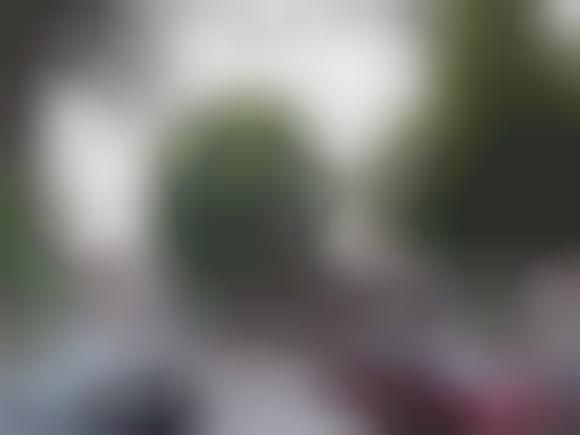The image is entirely blurry and out of focus, making it hard to identify the subject. At the center of the image, there is a green circular figure that is lighter at the top and darker at the bottom. A black band appears across the center of this figure, although it might be a photographic artifact. White surrounds most of this green circle, particularly at the top and left, possibly resembling the sky. The image also contains a dark object on the left that extends upward and arches to the right. On the right side, there's a larger green blob with some green extending from the top. The lower right corner shows a reddish highlight or patch, while the lower left contains something dark, likely black. The image features a combination of dark areas, shadows of light, and colors including white, green, and red amidst varying levels of blurriness, making it highly ambiguous and indistinguishable.